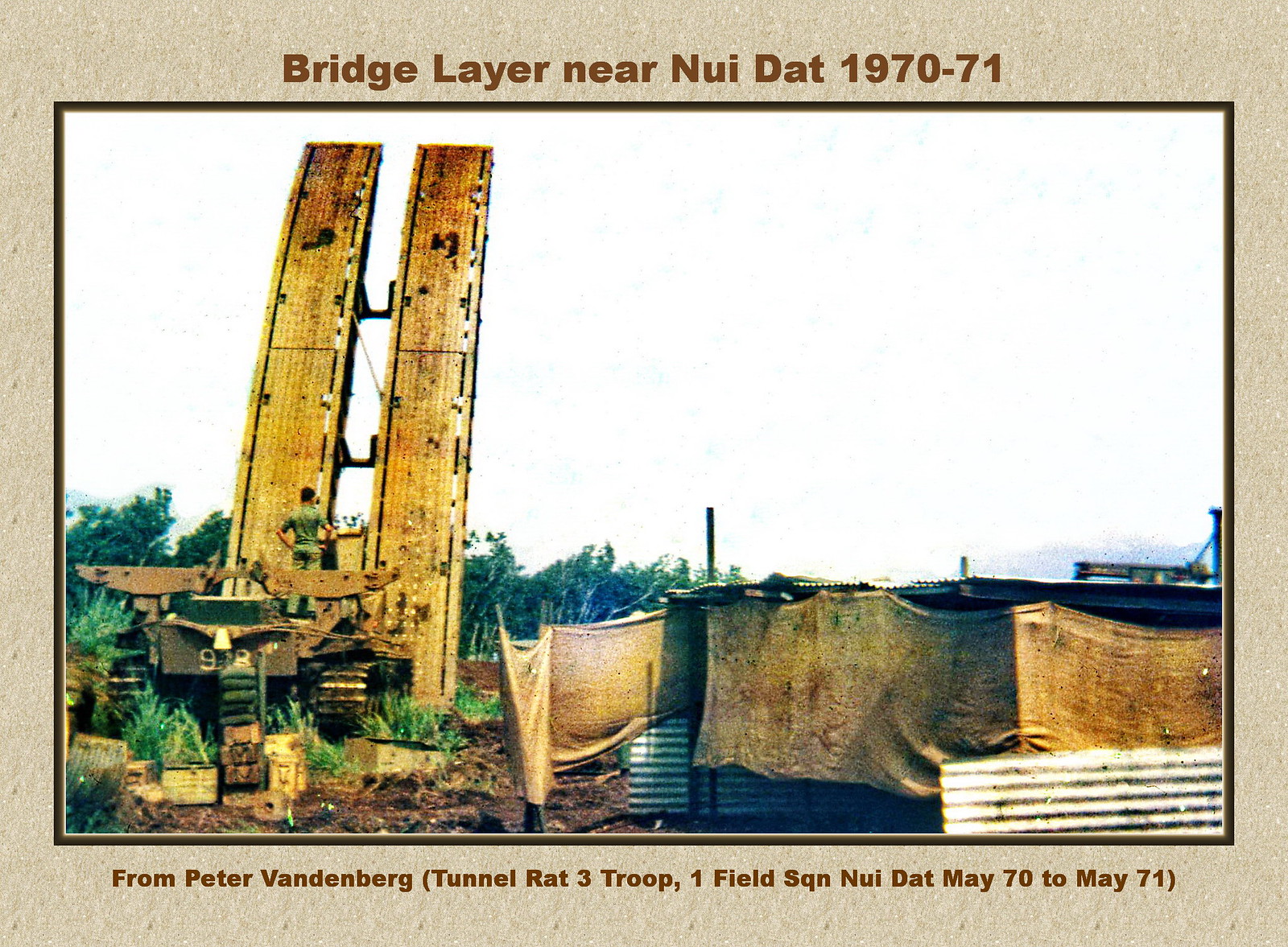The photograph, framed by a beige outline and a thin brown border, captures a moment from the Vietnam era, specifically near Nui Dat during 1970-71. At the top of the image, in brown lettering, it reads, "Bridge Layer Near Nui Dat, 1970-71," and at the bottom, it is attributed to Peter Vandenberg, with the text "Tunnel Rats 3 Troop, 1 Field Squadron, Nui Dat, May 70 to May 71." The scene is set outdoors during the daytime, under a partly cloudy sky. The central focus is a large piece of heavy machinery, likely a bridge layer, with part of a bridge suspended in the air on the left side of the image. A person in a green uniform stands in front of the machinery, back to the camera. To the right of the bridge layer, various materials and structures resembling metal sheets and fabric panels, possibly used as makeshift coverings or shelters, can be seen. The background features short trees and a dirt ground, characteristic of a construction site, with the main colors in the image being white, yellow, and green.